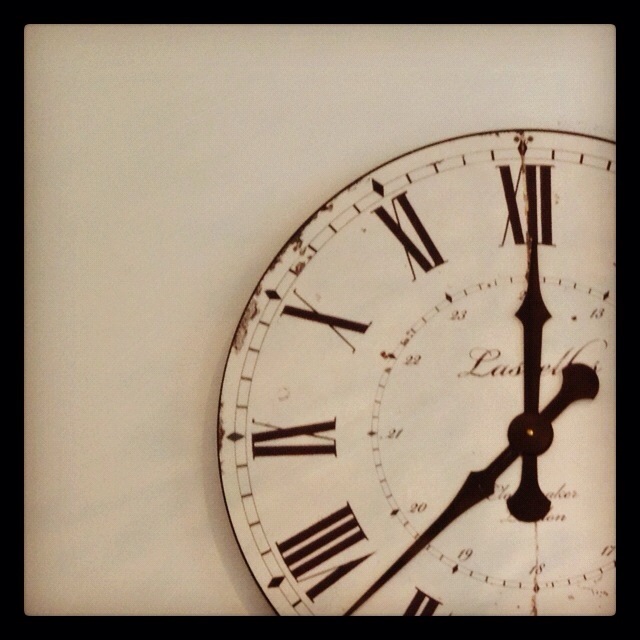This image features a photograph of a vintage round-faced clock positioned in the lower right corner, framed by a thick black border. The clock face, aged and showing signs of wear and rust, particularly around the 9 to 12 o'clock area, rests against a yellowish eggshell white background. The clock's outer edge is adorned with a thin strip of black metal. The face displays Roman numerals with dark brown accents, and the visible numerals range from XII to VII, with parts of the VI and the right side of the clock cut off. The inner ring of the clock includes a 24-hour scale with small numbers such as 23, 22, 21, and so on, while the outer ring features dashed lines indicating minutes and diamond-shaped marks for every five-minute interval. The clock's hour and minute hands, also brown, point to approximately 11:38, with the hour hand almost directly on XII, suggesting an inconsistency. Watermarks or marks further accentuate its aged appearance. In the center of the clock face, partially obscured cursive text suggests a manufacturer’s name, potentially "Lasell." The overall image’s aesthetic is completed by the contrast of the clock's beige and brown tones against the background and bordered frame.